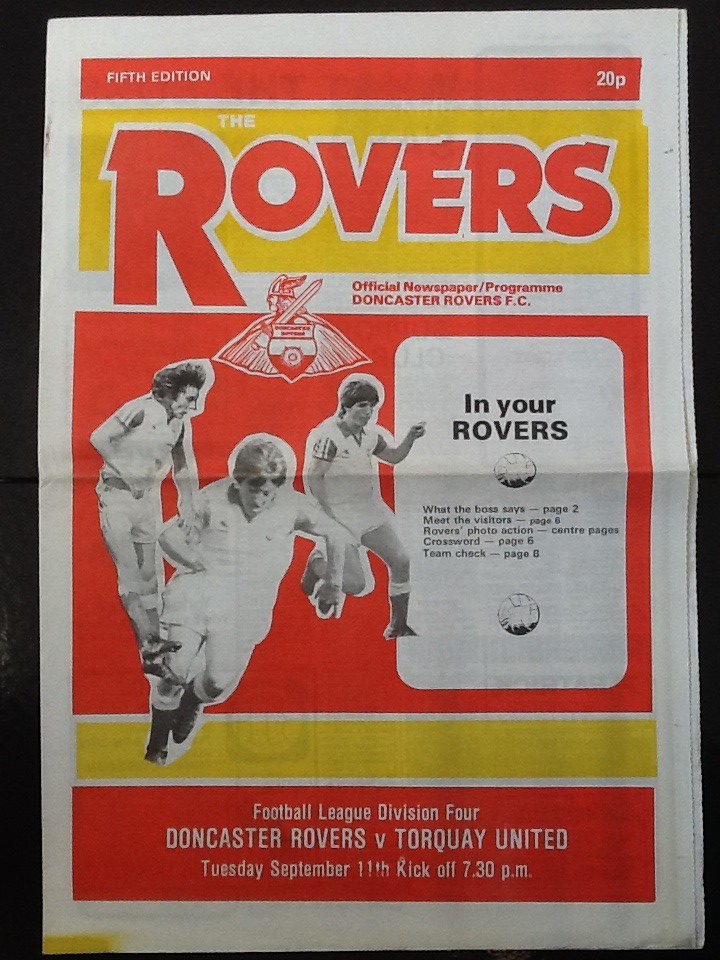This is the official cover of a program for a sporting event, presented on a white background with a black border accentuated by vibrant red, yellow, and black elements. Across the top, a prominent red strip extends from left to right, featuring bold white text in all capitals that reads "5TH EDITION" and "20P" in the right corner. Just below the red strip, a yellow banner and a large red letter "R" boldly stand out, with the word "OVERS" in red, outlined in white, and a small "V" placed above it. Under this, another white strip declares "Official Newspaper / Program" and identifies "Doncaster Rovers F.C."

A red box below this section showcases three separate black-and-white action photographs of soccer players, each outlined in white. Adjacent to these images is a white box, detailing various sections of the program with black text: "In Your Rovers, page 2," "Meet the Visitors, page 6," "Rovers Photo Action, center pages," "Crossword, page 6," "Team Check, page 8," and features a black-and-white soccer ball.

Further down, another yellow banner leads into the closing section of the cover, which consists of a red banner at the bottom proclaiming "Football League Division 4" and "Doncaster Rovers v. Torquay United." The event is scheduled for Tuesday, September 11th, with a kickoff time of 7:30 p.m. The program does not specify the year.